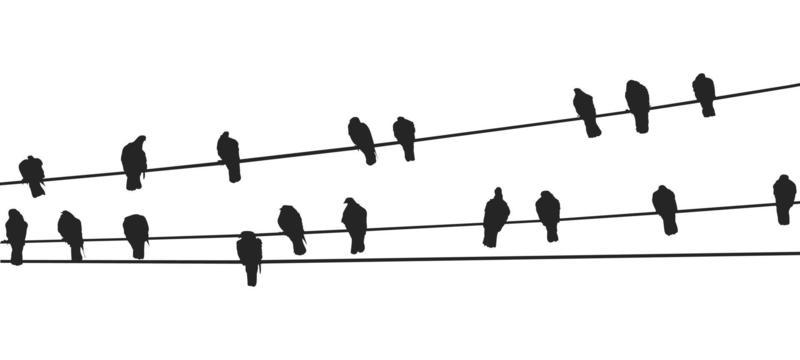This is a black and white illustration featuring a minimalistic design. Against a stark white background, three horizontal black lines, resembling electrical or power lines, span the width of the image. The top line has eight birds perched on it, while the second line down hosts nine birds positioned in various groupings: primarily three groups of three, with an additional bird on the far right. The third and bottom line holds a single lone bird. All birds are rendered in solid black silhouettes, devoid of any detailed features, emphasizing their shapes. The image is stripped of labels or any other colors, maintaining a simplistic yet evocative composition.